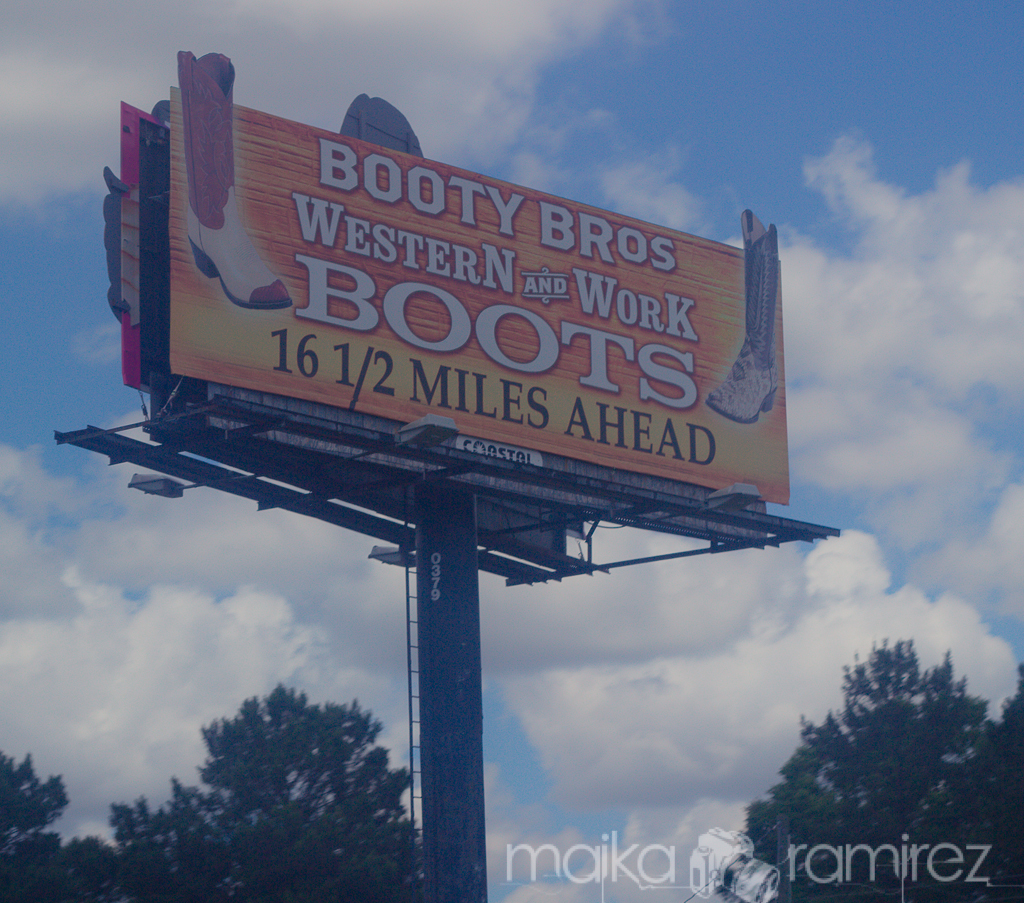The image showcases a towering highway billboard advertising "Booty Bros Western & Work Boots," located 16.5 miles ahead. The dual-sided sign—though only one side is visible in the picture—features an eye-catching, vibrant design dominated by warm orange and yellow hues. Prominently displayed on the sign are two large boots that extend over the edges, emphasizing the product being advertised. The backdrop of the scene includes a vivid blue sky filled with scattered clouds, through which patches of blue are still discernible. In the lower portion of the image, a line of trees is visible, providing a natural frame. The billboard is supported by a substantial, thick pole equipped with a secure ladder leading up to the sign, underscoring its formidable height and the accessible structure for maintenance.